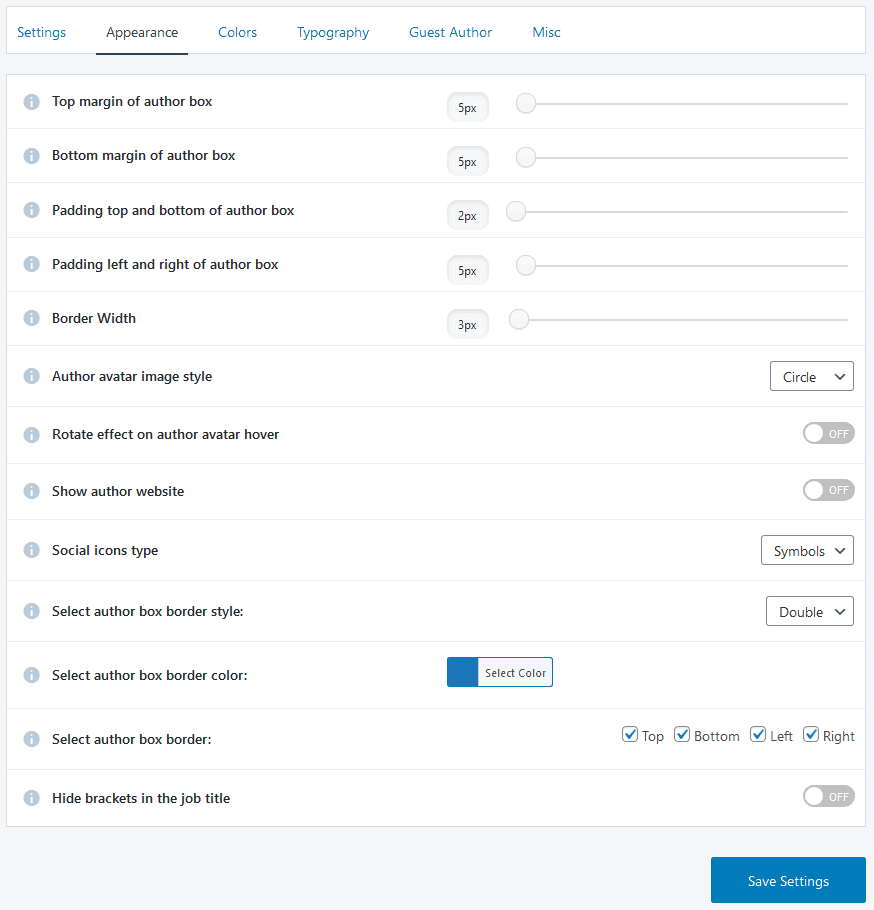The image depicts a vertically oriented rectangular box. At the top of the box, there is a white border with blue text displaying menu options labeled as "Settings, Appearance, Colors, Typography, Guest Author, and Miscellaneous." The "Appearance" option stands out, written in black and underlined.

Beneath this header, there is a series of rows extending from the top to the bottom of the box. Each row features a small information icon positioned to the left of its label, explaining various settings related to the author's box appearance. Some rows also include additional elements on the right-hand side, indicating adjustable parameters.

The first five rows are labeled:
1. "Top Margin of Author Box"
2. "Bottom Margin of Author Box"
3. "Padding Top and Bottom of Author Box"
4. "Padding Left and Right of Author Box"
5. "Border Width"

Each of these rows is accompanied by measurement fields on the right, specifying the dimensions.

Following these, the next section includes various style and functionality settings:
- "Author Avatar Image Style"
- "Rotate Effect on Author Avatar Hover"
- "Show Author Website"
- "Social Icons Type"
- "Select Author Box Border Style"
- "Select Author Box Border Color"
- "Select Author Box Border"
- "Hide Brackets in the Job Title"

This detailed list outlines the customization options available for configuring the appearance of the author's box.